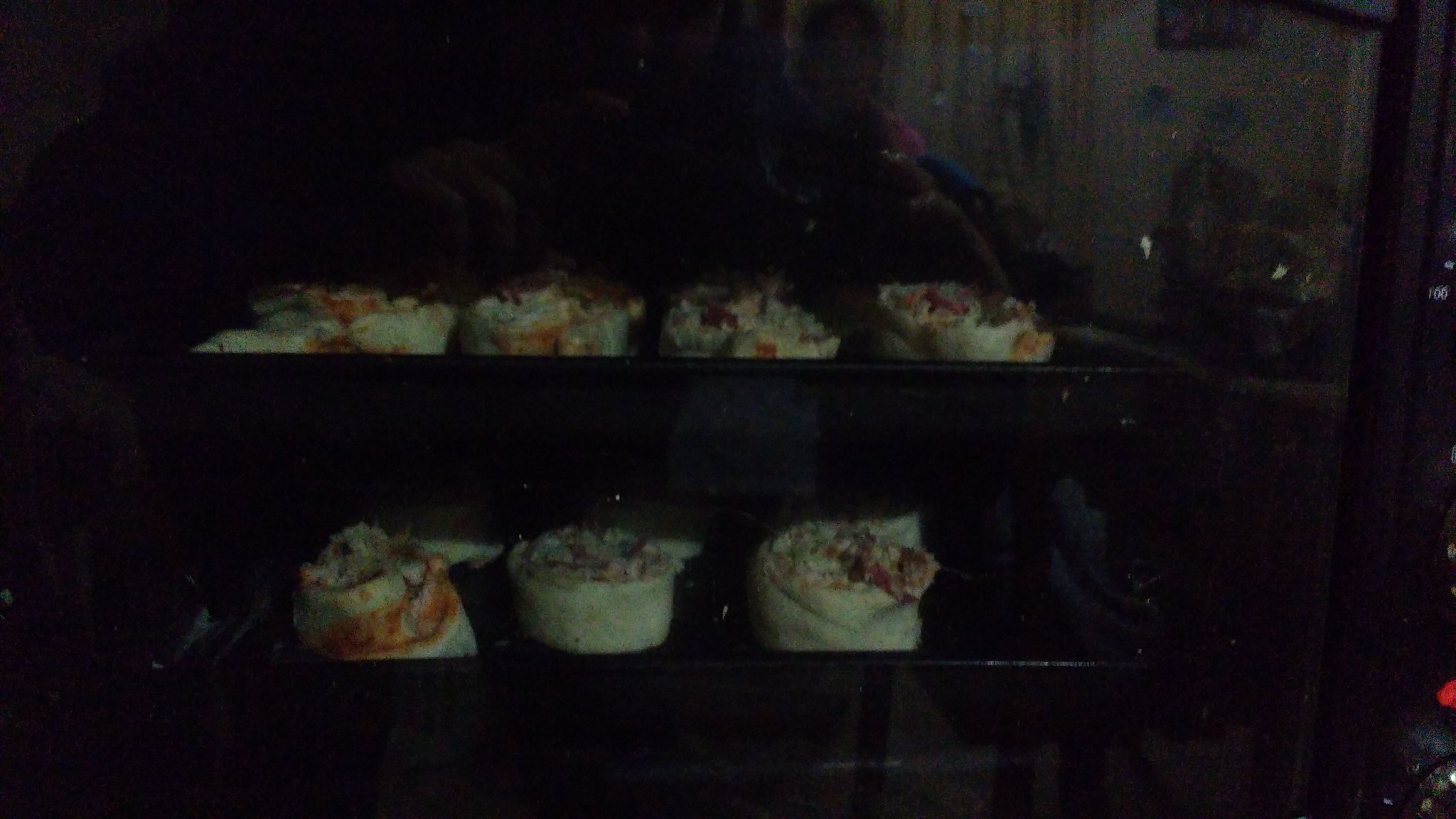The image is a highly underexposed and grainy landscape colour photograph, likely taken through the door of an oven since there is a glass reflection suggesting a room behind. Despite the low visibility, the photograph appears to show two dark, rectangular baking pans, possibly measuring around 13 by 9 inches each. Inside the pans, there are rows of food items resembling stuffed dough or pastry rolls, which look uncooked due to their pale, almost whitish-green appearance. The filling inside these rolls is indistinct due to the blurriness, but patches of red and chunky elements suggest a mix that could include tomato sauce and meat. There are two rows of these rolls: one raised in the bottom third of the image and a horizontal line of several more in the middle. The overall scene remains predominantly dark, with limited visible details, including a possible control dial or number on the right side hinting at the presence of an oven. The top of the image is almost entirely black, obscuring further details.